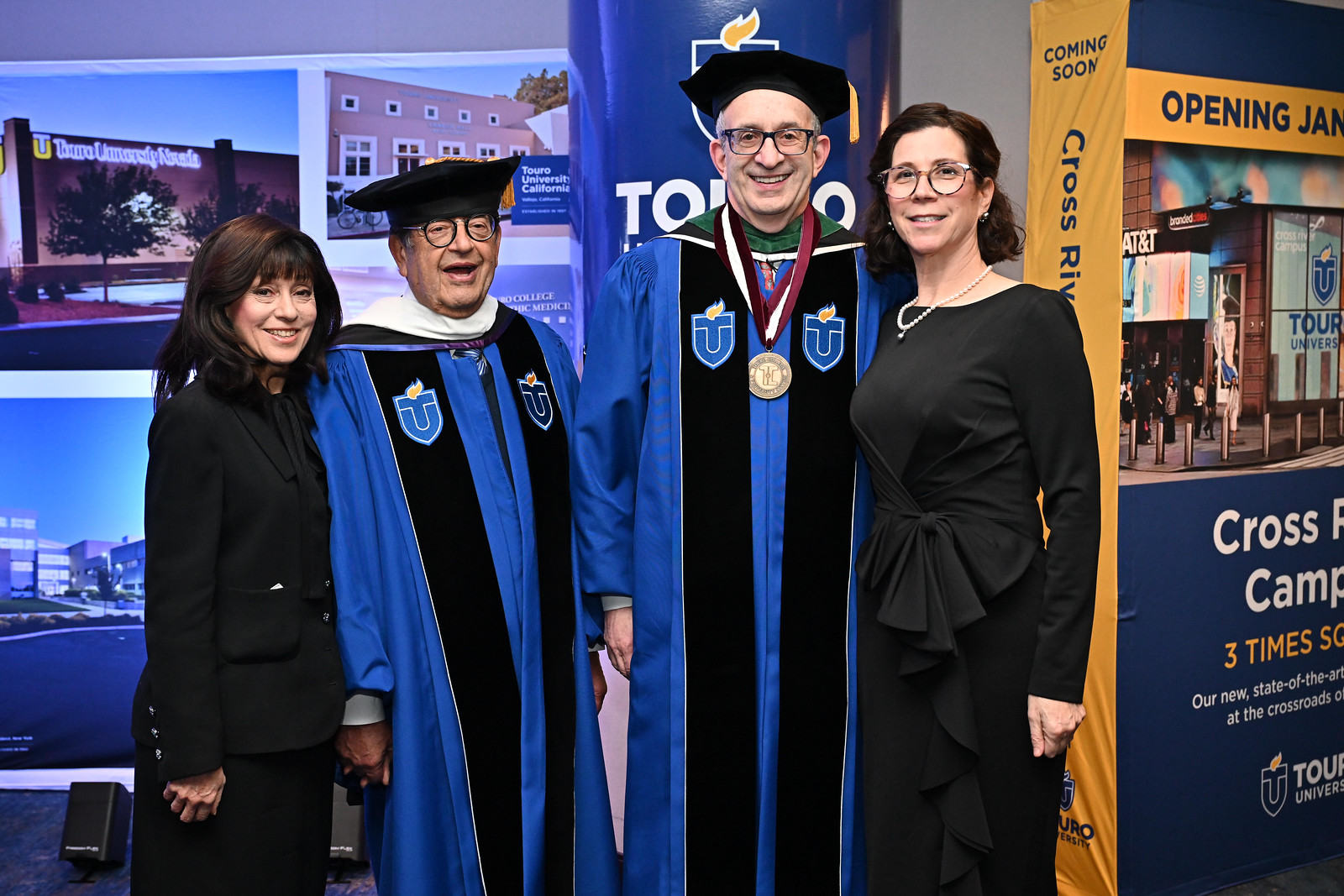This image depicts four individuals standing together at what appears to be a graduation ceremony at Touro University in California. The group consists of two middle-aged women and two elderly men, all of whom are white. The two men, positioned in the center, are wearing dark blue robes with black vertical stripes and matching black hats. They also have eyeglasses and are smiling. One of the men, distinguished by a gold medal around his neck, wears the robe adorned with a university emblem featuring the letters "T" and "U" accompanied by a torch. 

To the left of the men is a woman in a black blazer and pants with long black hair. On the right, another woman with brown hair is dressed in a black jacket and skirt, sporting glasses and a pearl necklace. 

The background showcases a campus scene with images of brick and white buildings near water. A blue banner with partial white lettering ("T-O") and other indistinguishable writing hangs behind them. Additional elements in the background include a blue and gold sign related to a campus tour and another with the text “Cross Camp” over a picture of a building, adding to the academic atmosphere.